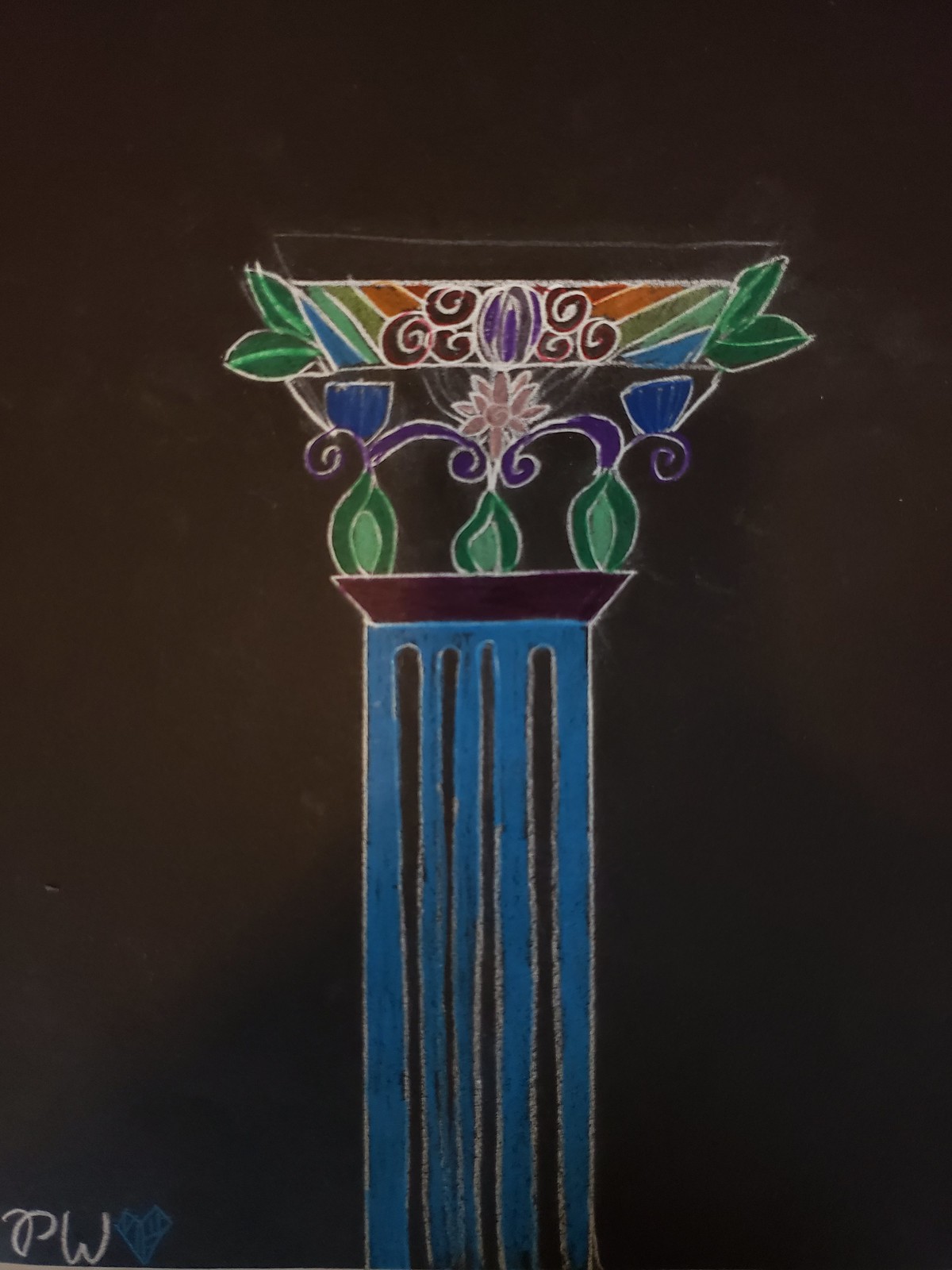An intricate illustration set against a stark black background features a prominent blue pillar at its center, adorned with four vertical dark lines. The pillar is capped with an angled structure that flares out to the sides before straightening across the top. Atop this structure sit three teardrop-shaped elements, each displaying a gradient from dark green on the outside to light green on the inside. Emerging from these teardrops are three distinct flowers: the outer two bear rough tulip-like blue blooms, while the central teardrop boasts a lush, many-petaled pink flower. Crowning the composition, vibrant rainbow-colored rectangles extend outward from the sides. Adding a final touch of natural elegance, green leaves elegantly frame the entire piece.